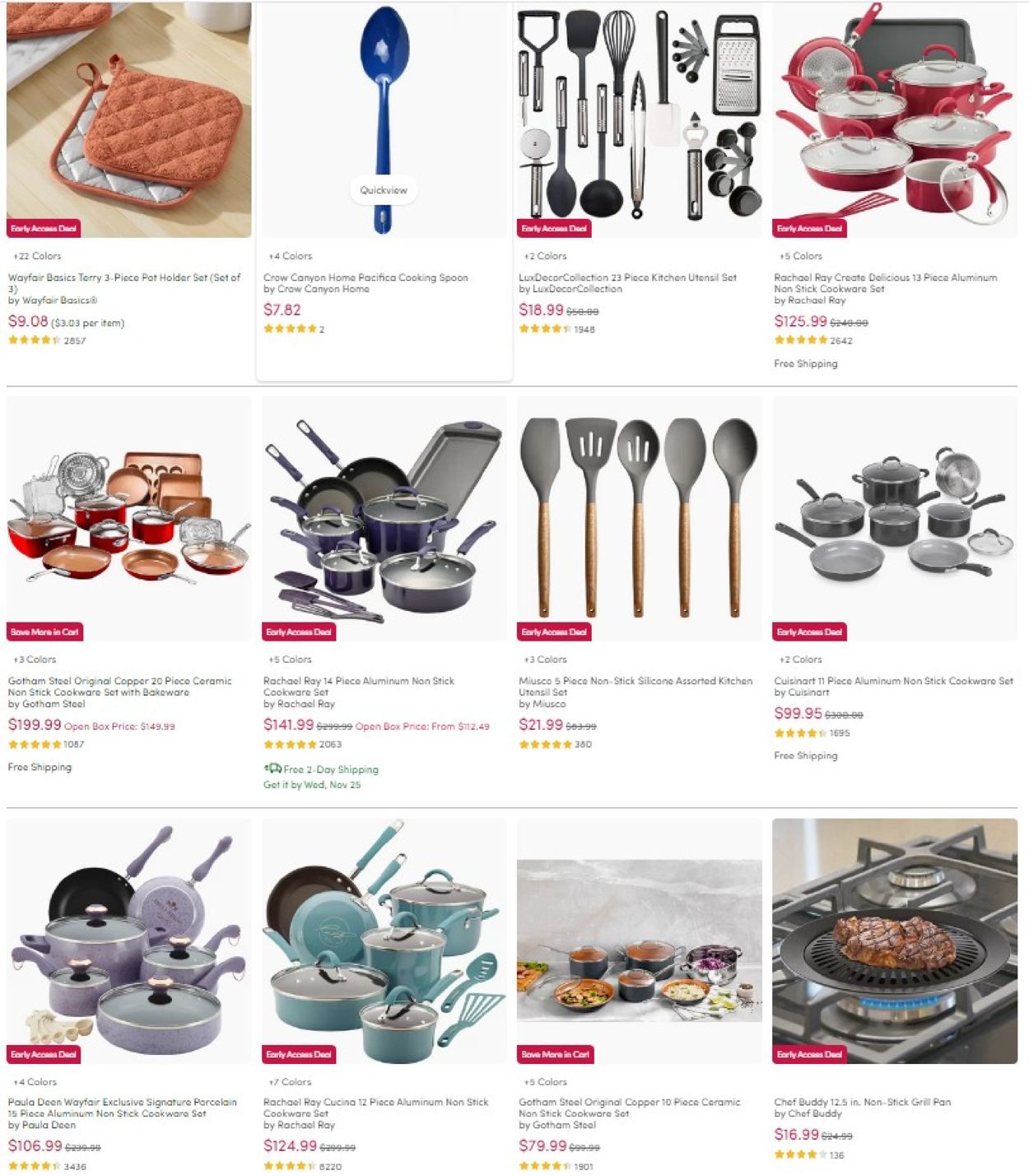The image showcases a grid of kitchen products available for sale on Amazon, organized into three rows of four items each against a white background.

**Top Row:**
1. **Oven Mitts** - Priced at $9.08, these mitts are positioned in the top-left corner.
2. **Blue Spoon** - To the right of the oven mitts, priced at $7.82.
3. **Kitchen Utensil Set** - A package deal of various utensils, available for $18.99.
4. **Cookware Set** - A comprehensive set of kitchen cookware, priced at $125.99.

**Middle Row:**
1. **Cookware Package Deal** - Starting from the left, this package is priced at $199.99.
2. **Gray Cookware Set** - To the right of the cookware deal, available for $141.99.
3. **Five Kitchen Spoons and Spatulas** - Priced at $21.99, this set includes various spoons and spatulas.
4. **Another Cookware Set** - On the far right, priced competitively at $99.95.

**Bottom Row:**
1. **Cookware Set** - Positioned on the left, priced at $106.
2. **Light Blue Cookware Set with Gray Tops** - This colorful set is available for $124.99.
3. **Cookware Set** - Another cookware set priced at $79.99.
4. **Oven Burner Item** - Located on the far right, priced at $16.99.

This detailed layout allows for easy comparison of prices and types of kitchen products available.